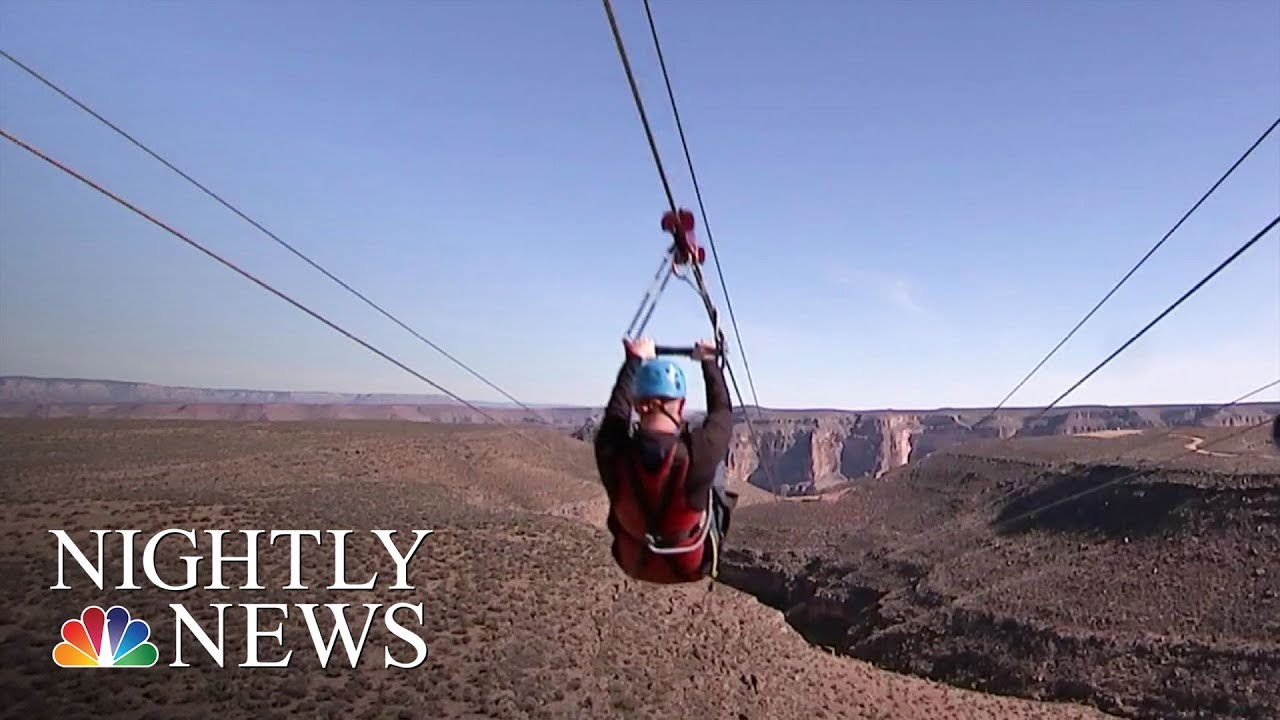A man is captured suspended mid-air while ziplining across the expansive Grand Canyon in this vivid color photograph. Positioned centrally in the image, he grips a triangular support bar and is outfitted in a maroon shirt and a light blue helmet, with essential safety gear visible. The photo shows three ziplines converging diagonally from the top towards the center, enhancing the sense of adventure. Below, the Grand Canyon presents a patchy mosaic of brown and gray terrain, amplified by the clear blue sky overhead. The left side of the image features the white text "Nightly News" accompanied by the colorful NBC peacock logo, contributing to a dynamic blend of sports and outdoor adventure.